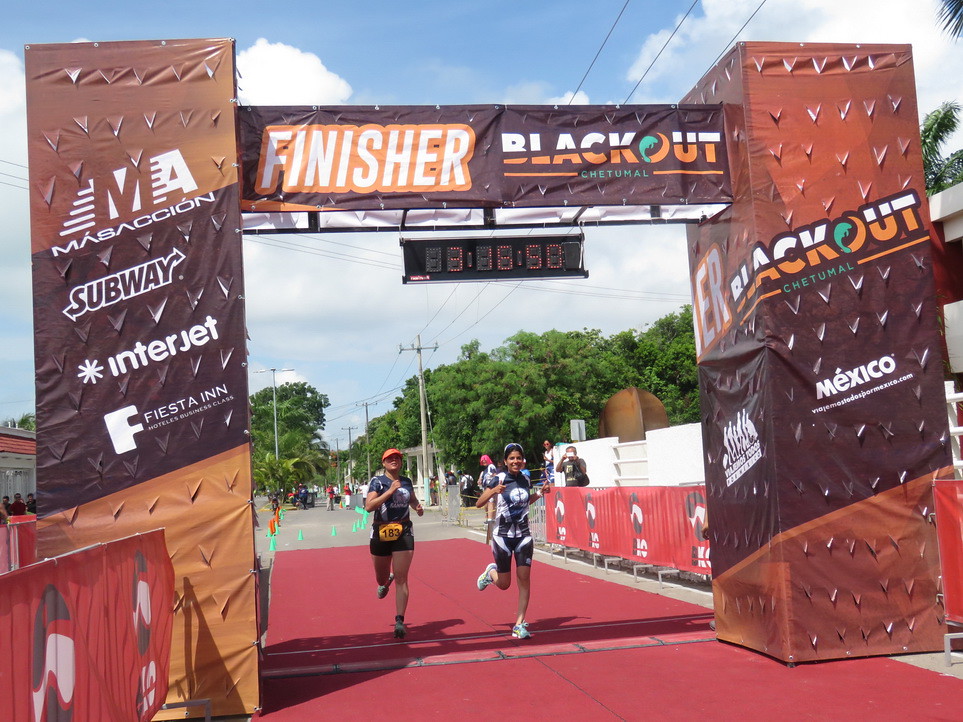The image depicts a vibrant outdoor scene at a running competition, where two female runners are about to cross the finish line, marked by a prominent gate with a sign reading “Finisher Blackout Chetumal, Mexico.” The finish line is adorned with a red carpet that accentuates the moment of triumph. A digital clock above the gate displays a time of 3:16:50. The runner on the right, dressed in black and white biker shorts and a tight shirt with her hair pulled back, is smiling as she approaches the finish. Her companion on the left, wearing black shorts and an orange hat, sports a yellow bib at her waist numbered 183. The background features a blue sky with scattered white clouds, distant green trees, and several other participants further down the course. The scene is surrounded by fencing draped in red with multiple sponsor advertisements, including Subway, Interjet, and Fiesta, adding to the event’s lively atmosphere.